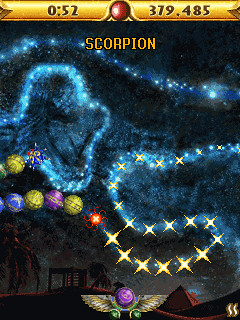Screenshot of a computer game interface. At the top of the screen is a gold bar displaying the time "0:52" on the left and a red circle in the middle. To the right of the red circle is the score "379.485" in large gold text, followed by the word "Scorpion" in the same gold hue. 

The main portion of the screen is predominantly dark gray, intersected by several visually striking elements. A series of deep blue lines, dotted with light blue lights, traverse horizontally from the left side and gently curve downwards towards the right. Within this network of blue lines, there appears to be a vaguely discernible figure, possibly a person, enclosed in a glowing blue halo.

On the right side, another blue line appears, adding symmetry to the design. Below these elements, a pathway of gold X's is visible, beginning small and gradually increasing in size. The path formed by the X's transforms into a red squiggly line midway through.

Further down the screen, a sequence of colored balls—gold, purple, gold, and blue—forms a curving trail that momentarily disappears off-screen before reappearing with another gold ball. Nearby, a small bluish-red creature adds to the dynamic scene, emphasizing the intricate and lively nature of the game interface.